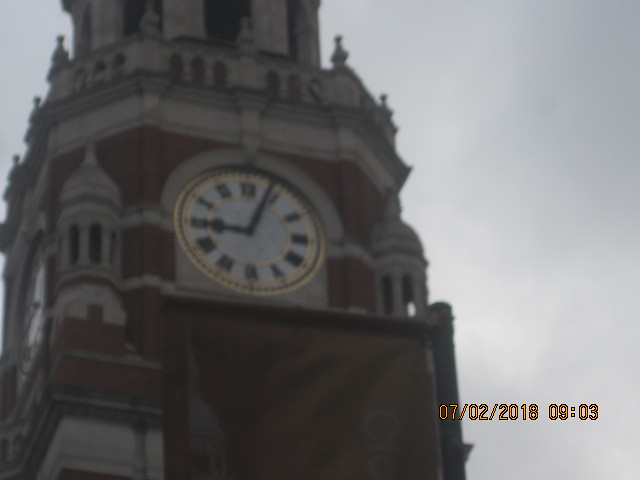This detailed image captures a grand clock tower integrated into the side of a majestic building. The clock is positioned approximately one-third from the bottom, angled to the right. The upper part of the right side of the image transitions into a blue sky, hinting at impending rain. The top part of the building showcases gray pillars with two small black slots resembling doorways at its center. 

In front of these pillars, a concrete railing features three slits in each segment, adorned with small statues atop the outer edges of these openings. Below this railing is a gray brick border. Flanking the building are two columns with slit openings, peaking at the top. Between these columns, the red brick facade is highlighted by a gray half-circle arch, housing the prominent clock.

The clock itself is white, bordered by gold trim, and features black Roman numerals. Both the hour and minute hands are black, though the hour hand is short and thick, while the minute hand is long and thin. Directly beneath the clock, a red flag hangs on a black pole extending towards the right. Additionally, yellow lettering in the bottom right corner displays the date "07/02/2018" and the time "9:03".